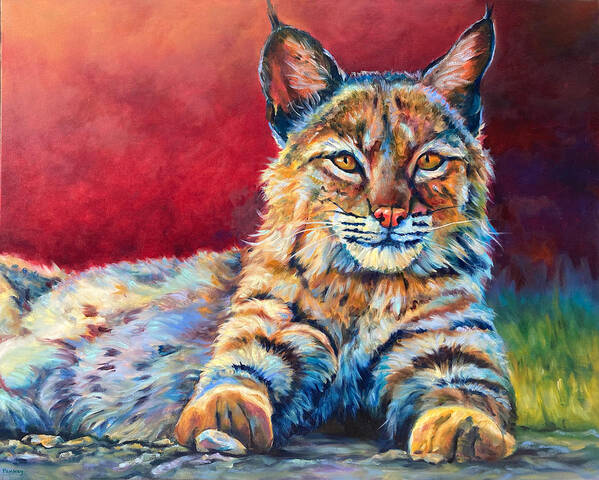The artwork is a detailed drawing of a cat situated in an outdoor setting. The cat is predominantly orange and black with striking orange eyes and an orange nose. Its pointy ears, outlined in black, have striking red interiors. The cat's white whiskers, extending from the black portion of its face, are prominent. The feline is captured in a seated position with its two front paws visible, colored orange at the front. Its body is turned to the left but the head is turned towards the viewer, giving a partial profile view. 

In the background, a dramatic red sky transitions from orange and red in the top left corner to a darker red in the top right. This intense backdrop contrasts intriguingly with the gray rocky surface in the foreground and a patch of green and yellow grass to the right of the cat. The cat's tail curls into the lower left corner of the image. The overall palette includes additional vibrant hues, subtly suggesting the cat might have some rainbow-like accents, particularly reflecting various shades such as purple, blue, yellow, and white interspersed in its fur. The composition is vivid and rich in color, enhancing the cat's dynamic presence against the stark, striking background.